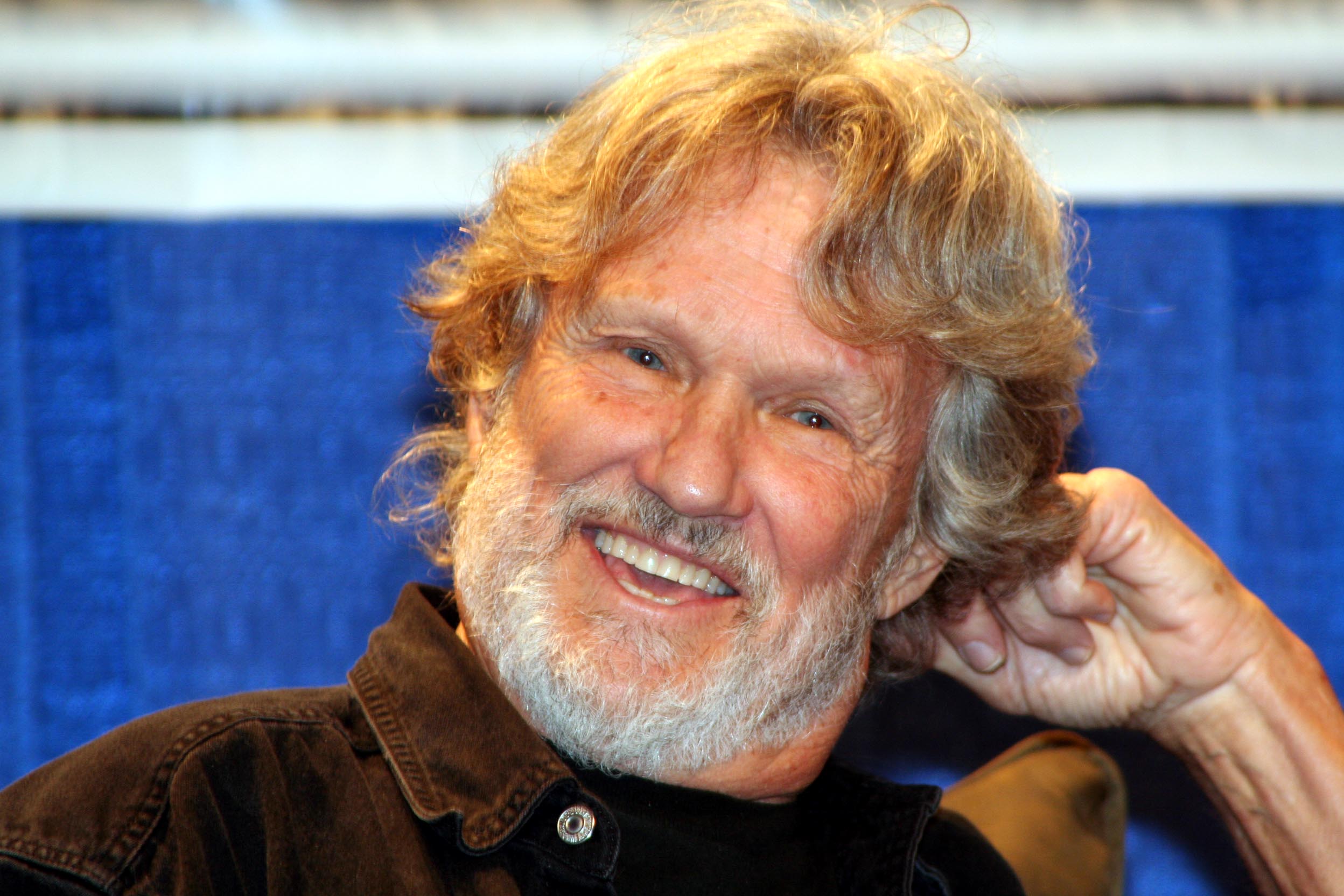In this image, the background features a striking contrast with its upper section being a blurred white strip stretching horizontally from left to right, and the lower portion a solid blue. The main subject of the photograph is an elderly man with a prominent presence. His long, flowing hair is a mix of tan, blonde, and grey hues, complementing his distinguished appearance. His facial hair is equally striking, with a thick, silver moustache and beard. The man is dressed in a unique black denim collared shirt, adorned with a noticeable silver button on the collar. He is captured in a moment of apparent contentment, resting his head on one fist while sporting a big, jolly smile. The overall ambiance of the image exudes warmth, character, and a sense of joyful reflection.